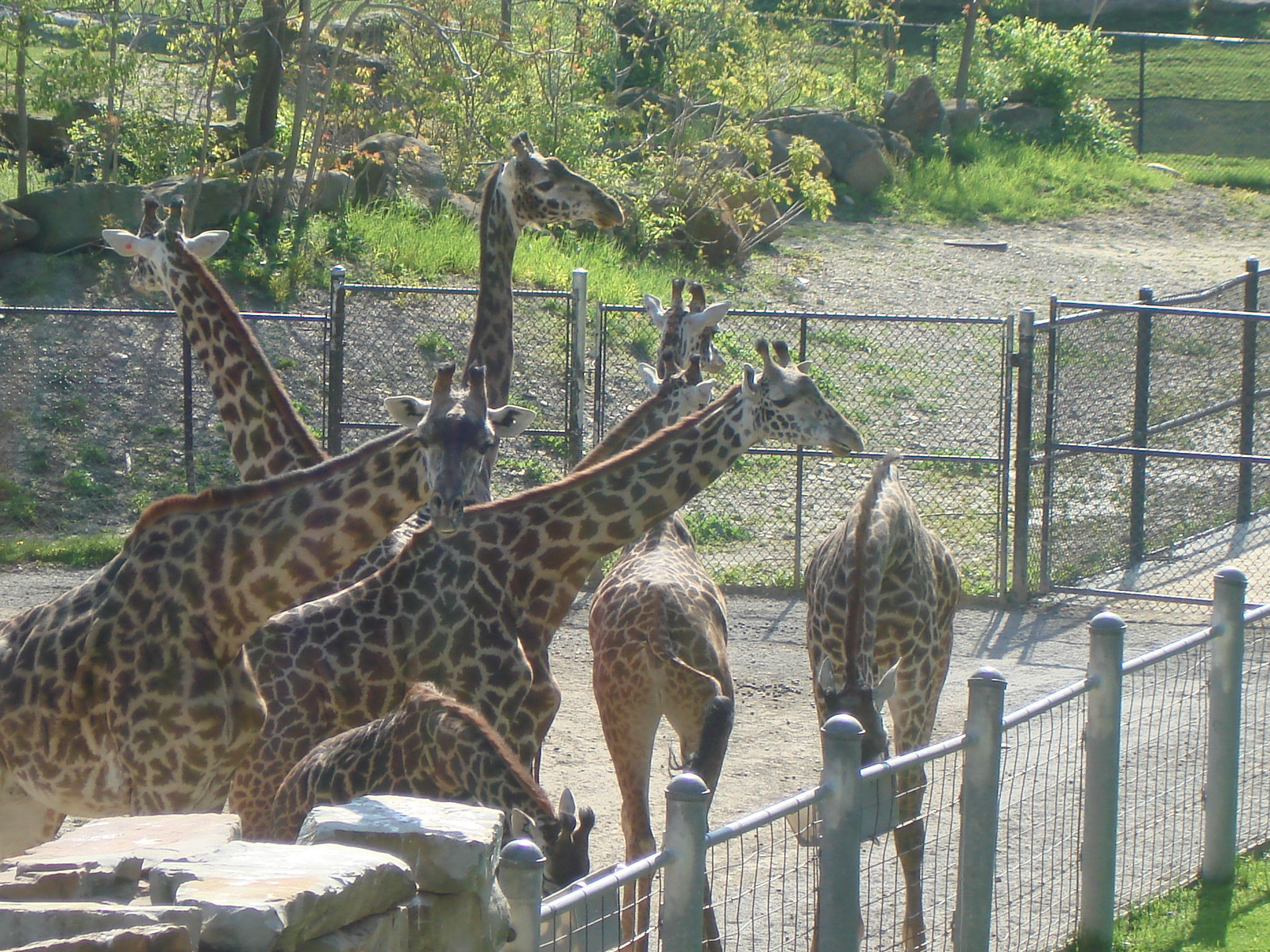This color photograph captures a group of giraffes within a chain-link enclosure, potentially at a zoo or a sanctuary. The enclosure is reinforced by metal posts every four feet, and the ground inside is hard and brown, contrasting with the greener landscape beyond. The background features a grassy area with trees and various plants. In the middle of the fence, there is a gate likely designed to allow the giraffes access to this more verdant section. 

In the enclosure, there are seven giraffes, making it somewhat difficult to count them precisely due to their intertwined necks as they huddle together. The giraffes vary in height, suggesting a mix of adults and younger ones. Among them, one giraffe looks directly at the camera, two gaze off to the side, two towards the grassy enclosure, and a couple have their heads lowered, seemingly investigating something on the ground. These majestic animals, with their long necks rising about three feet above the fence, are a striking sight, presenting a tableau of curiosity and grace as they peer out in different directions.